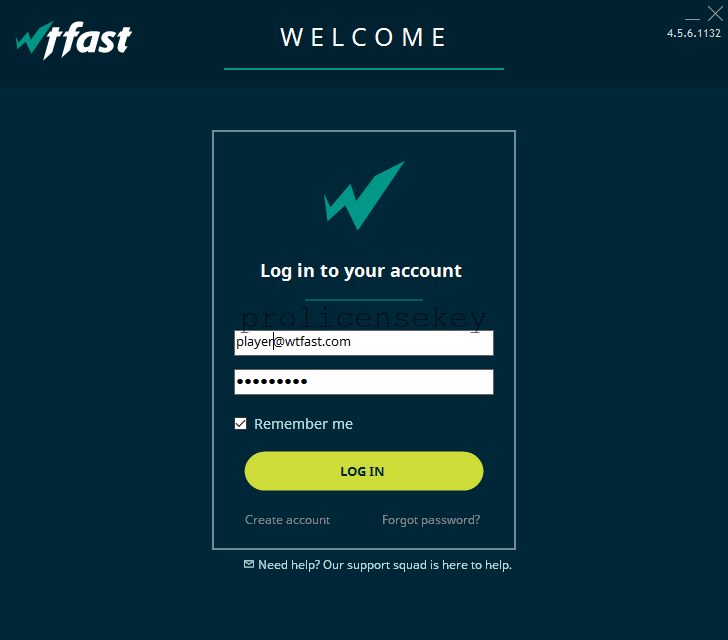This screenshot features the WTFast application, likely captured on a desktop given the close and minimize icons located at the top-right corner of the screen. Displaying version 4.5.6.1132 of the app, the overall background is a dark teal or deep blue color. Prominently placed at the top is a "Welcome" message in white text, underlined in green. 

On the left-hand side, the WTFast logo is displayed, with 'W' in green and 'TFast' in white. The central focus of the screenshot is a small login window. At the top of this window, the logo is either repeated or positioned prominently, followed by the text "Login to your account," also in white and underlined in green. 

The login interface includes fields for an Email ID—pre-filled as player@wtfast.com—and a password. Beneath these fields lies an option to "Remember Me," with the "Login" button, colored in green, just below. Below the login button, there are options to "Create Account" on the left and "Forgot Password" on the right. At the very bottom of the window, the text reads, "Need help? Our support squad is here to help," ensuring users have access to assistance if needed.